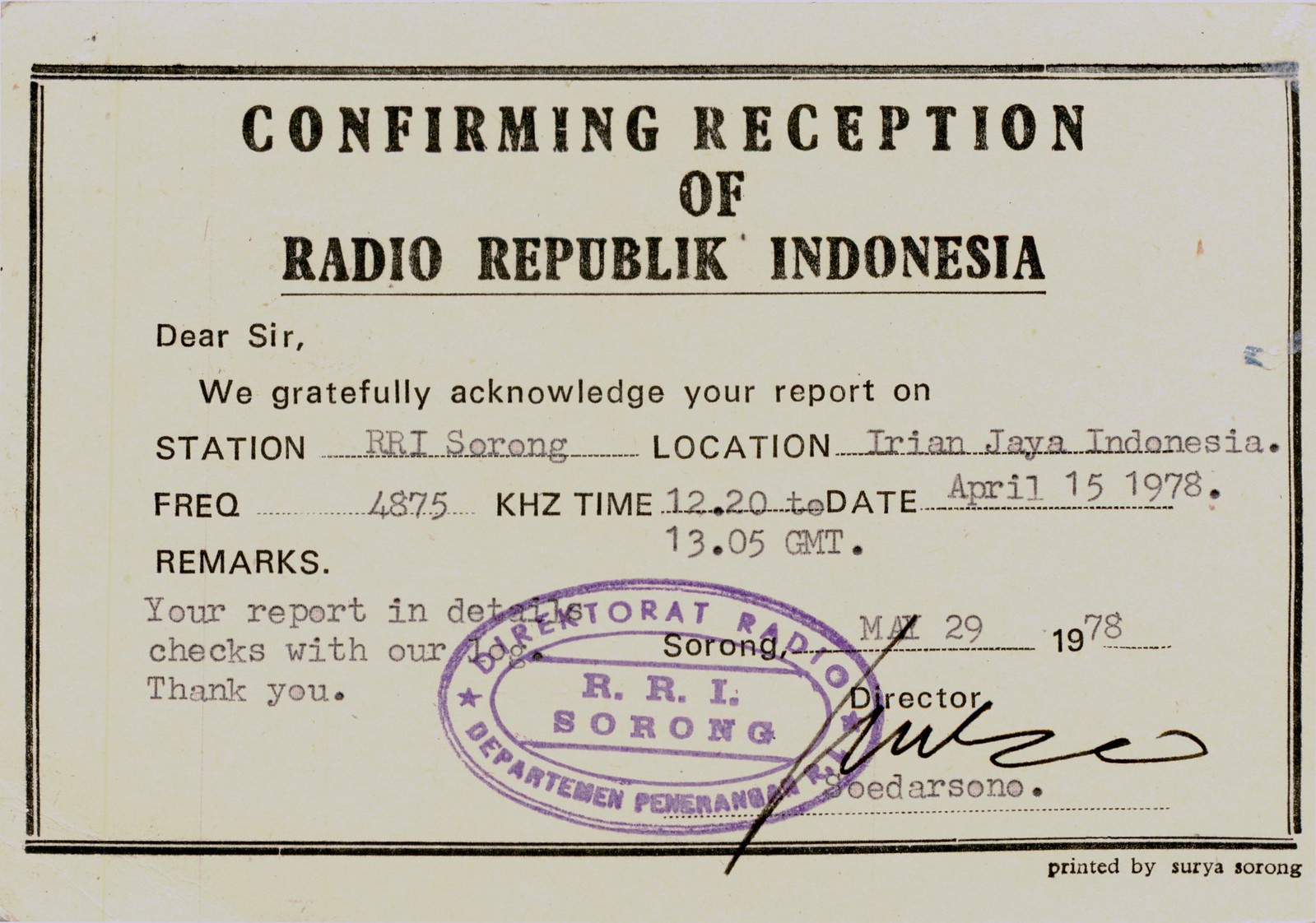This is a detailed photograph of an official acknowledgment certificate from Radio Republic Indonesia, formatted in a horizontally aligned rectangle. The certificate has a grayish-white background with black text and an official purple oval stamp. At the top, centered in bold, the text reads "CONFIRMING RECEPTION OF RADIO REPUBLIC INDONESIA," with "Radio Republic Indonesia" in a slightly darker, bold font and underlined. Below this, the text in a simpler font begins with "Dear Sir," acknowledging a report submission. Specific fields are filled in, including "Station: RRI SORONG," "Location: ARIAN JAYA, INDONESIA," "Frequency: 4875 KHz," "Time: 1222-305 GMT," and "Date: April 15, 1978." Remarks indicate the report's accuracy, stating "YOUR REPORT IN DETAIL CHECKS WITH OUR..." followed by a thank you note. The certificate is dated "May 29, 1978," signed by the Director, with the typewritten name "BETTER OUR SONO." The distinctive purple stamp bears the text "TOROTS RADIO" with initials "RRL" and "SORONG," along with stars and the department name, confirming its authenticity. The certificate was printed by Surya Sarong.